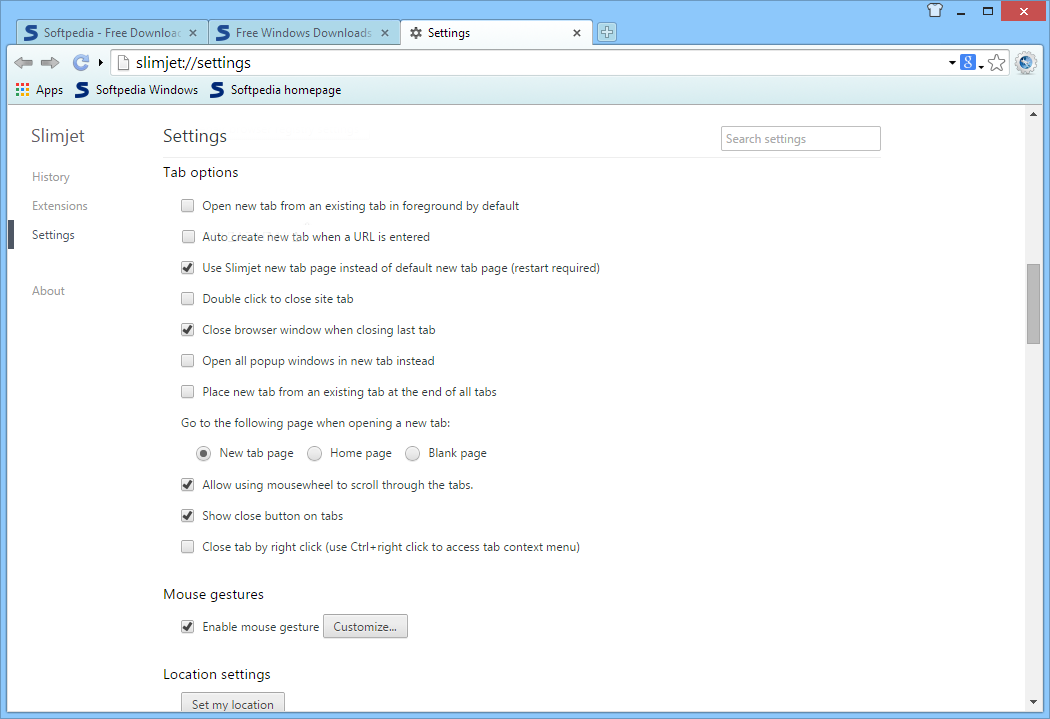The screenshot captures a window, likely from an older Microsoft browser such as Edge or Internet Explorer. The top of the window features a baby blue background. On the right side, there is an outline of a t-shirt and a black square with a white 'X' and a red rectangle. Below this, three links are open: two of them have an 'S' icon labeled "Softpedia, free download," and the third reads "free Windows downloads."

The system settings tab is also open, displaying in white with black text. There's a URL visible: 'SlimJet://settings,' indicating settings for the SlimJet browser. On the left-hand side, navigation options include SlimJet, history, extensions, settings, and about. The settings tab is active, showing various browser configuration options.

These options include:
1. Use SlimJet new tab page instead of the default new tab page (restart required).
2. Close browser window when closing the last tab.
3. New tab page settings.
4. Allow using the mouse wheel to scroll through tabs.
5. Show close button on tabs.
6. Enable mouse gesture (currently turned on).

Overall, this image provides a detailed look into the SlimJet browser settings and some open links for downloading free Windows software.